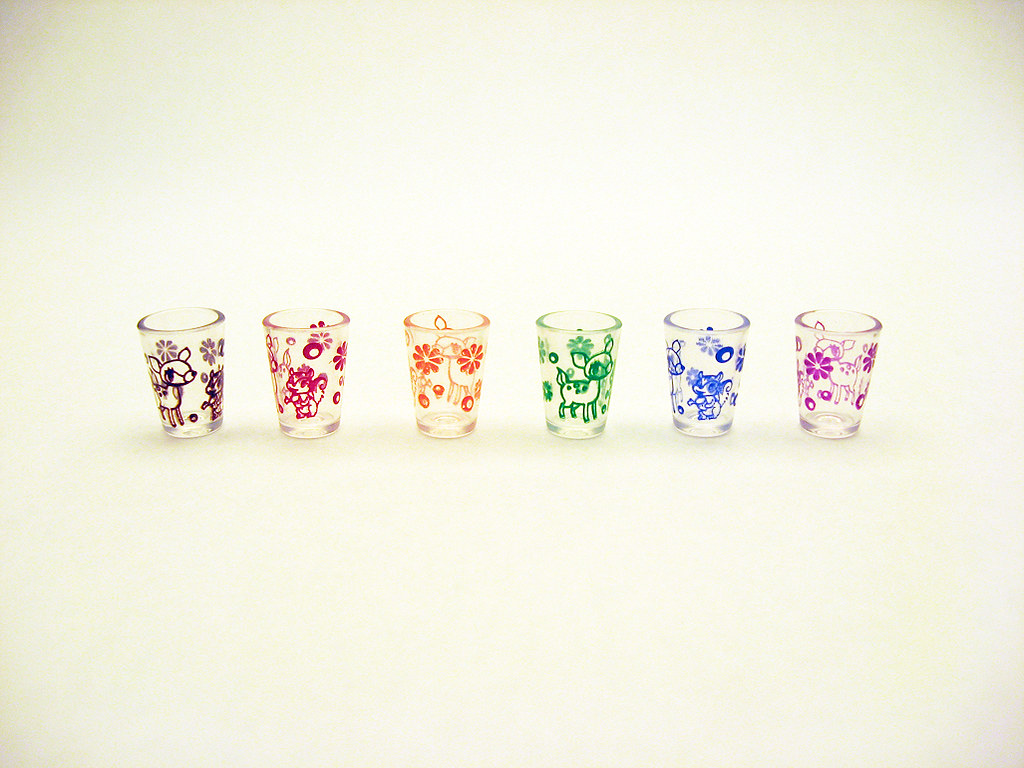The image depicts six clear shot glasses arranged in a straight horizontal row, each adorned with whimsical, colorful patterns against an off-white background that darkens towards the corners. The designs on the glasses are consistent, featuring intricate motifs of flowers, bubbles, a deer with big eyes and long eyelashes, and a squirrel facing the deer, though the colors and orientation of the designs vary. From left to right, the shot glasses display the following designs: the first has a black design with flowers and a fawn; the second features maroon patterns of a squirrel, flowers, and bubbles; the third is clear with orange designs showing bubbles, flowers, and a fawn visible through the glass; the fourth is green with the same fawn design; the fifth is blue, with partial views of the fawn and squirrel; and finally, the sixth shot glass has a purple floral design with the deer visible on the far side. Each glass is spaced about an inch apart, enhancing the showcase of their unique, yet cohesive designs.